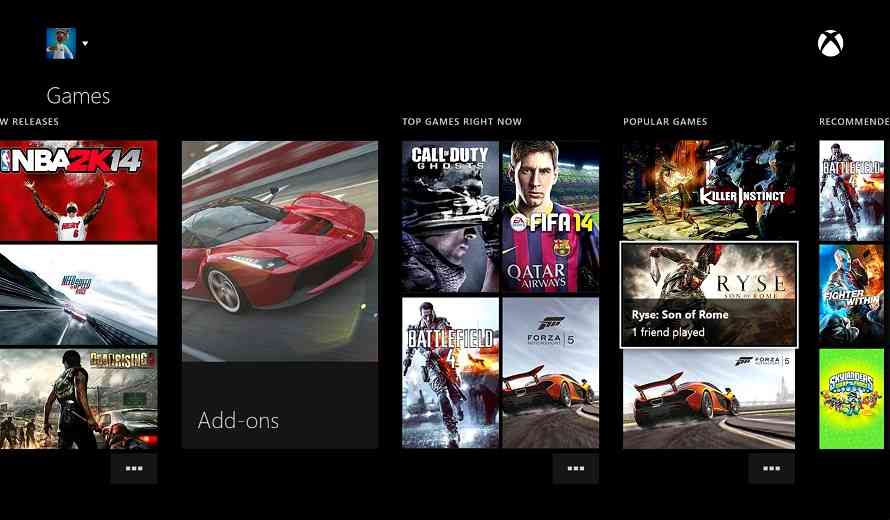This screenshot, taken from the Xbox website's games page, features a sleek black background with a minimalist design. At the top of the page, there is a header that includes a profile icon accompanied by a drop-down symbol. Beneath the header, the word "Games" is prominently displayed in white against the black backdrop. The content on the page is organized into several sections for ease of navigation.

The first section is labeled "New Releases" and showcases four different game cover images. Among them, "NBA 2K14" is clearly visible, while the titles of the other three games are not easily discernible. Adjacent to this section is a small rectangle with white text labeled "Add-ons."

The next section, titled "Top Games Right Now," highlights popular games such as "Call of Duty," "FIFA 14," "Battlefield," and "Forza." Each game is represented by its cover art.

Following that, another section titled "Popular Games" is displayed, leading into the "Recommended" section. Throughout the page, each game is visually represented by its associated cover art, providing a vibrant and engaging overview of available and trending games.